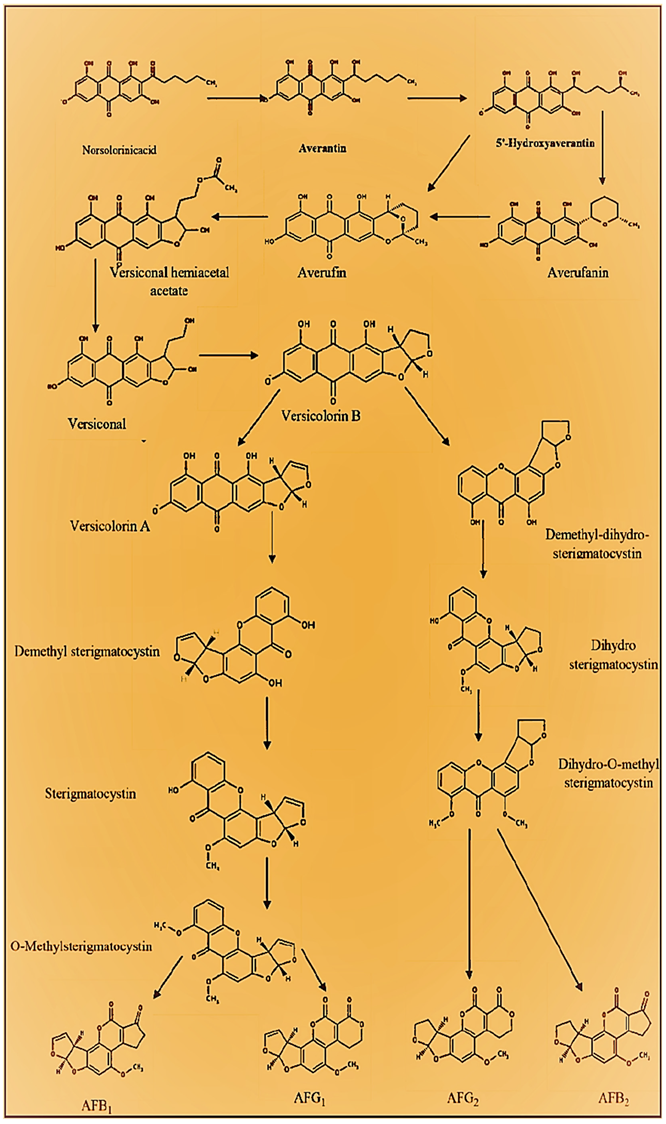This image is of a detailed diagram set against a yellow background, showcasing the progression of various organic chemistry compounds. It appears to be from a textbook or research paper, depicting 19 chemical compounds in total. The compounds are organized into a flowchart with arrows indicating the transitions between them. At the top, there are three compounds, followed by subsequent rows of three, two, two, two, and finally a row of four compounds at the bottom. The compounds are primarily made up of three to five hexagonal modules, with O or OH groups labeled at various corners. The four compounds at the bottom are labeled AFB1, AFG1, AFG2, and AFB2. The diagram illustrates the potential transformations that occur when specific reagents are added or removed from these compounds.